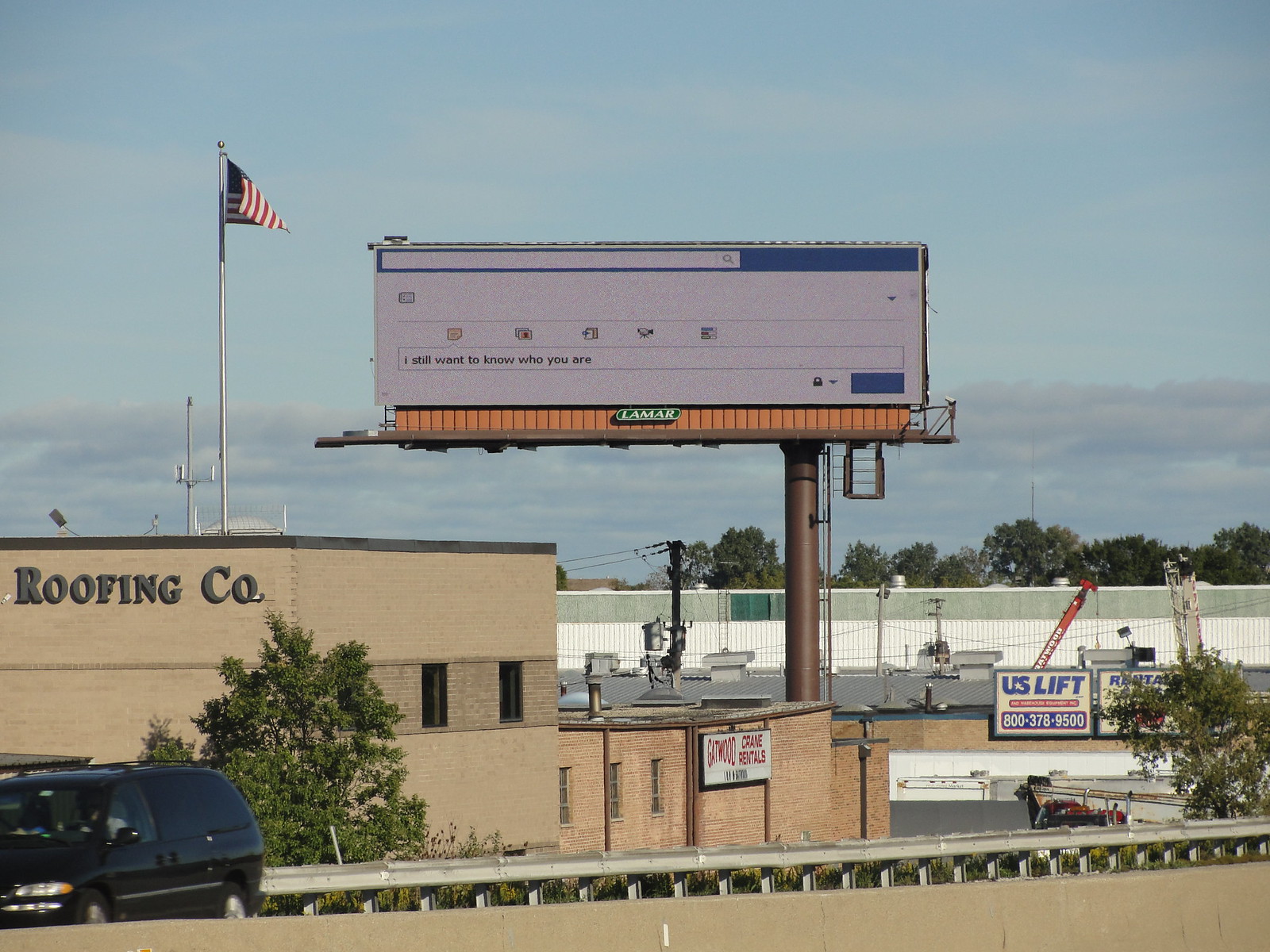This landscape-oriented photograph captures a bright, sunny afternoon with blue skies dotted by a few low-hanging clouds. The scene is dominated by a prominent tan-colored building with the label "Roofing Company" in gray letters. Above this building, an American flag flutters from a tall metal pole. To the left, there is a gray pillar, and near it, a black minivan drives in the opposite direction of the photographer's perspective. To the middle right of the frame stands a tall digital billboard displaying the message, "I still want to know who you are," reminiscent of a search engine query. Additional elements in the image include distant trees, another large building, and two cranes situated near the main building. In the lower right corner, text on the billboard mentions "US LEFT" alongside a phone number, 800-378-9500.